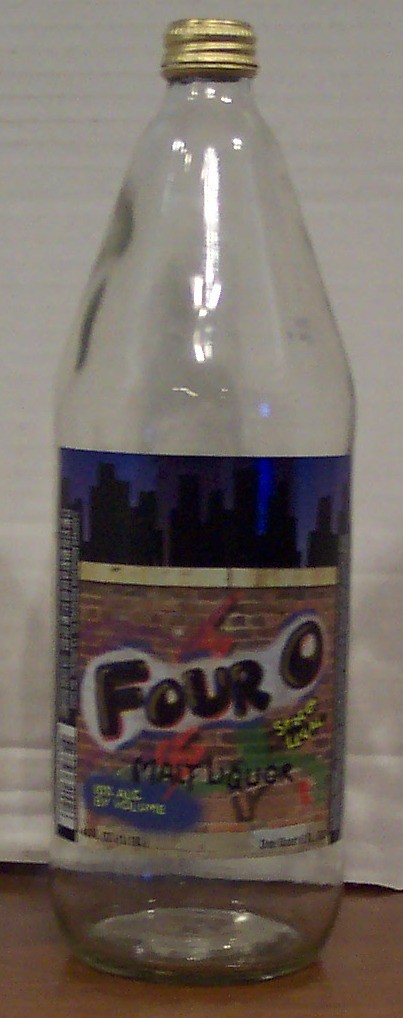A close-up image captures an empty bottle of 4-0 malt liquor. The bottle, photographed with what appears to be an older or lower-quality camera, features a golden screw cap and a label designed with a nighttime cityscape motif. Silhouetted buildings transition into a brick wall, where "4-0" and "malt liquor" are displayed in a graffiti style, accompanied by other indistinct elements. The bottle rests on a hardwood floor beside a white wall.